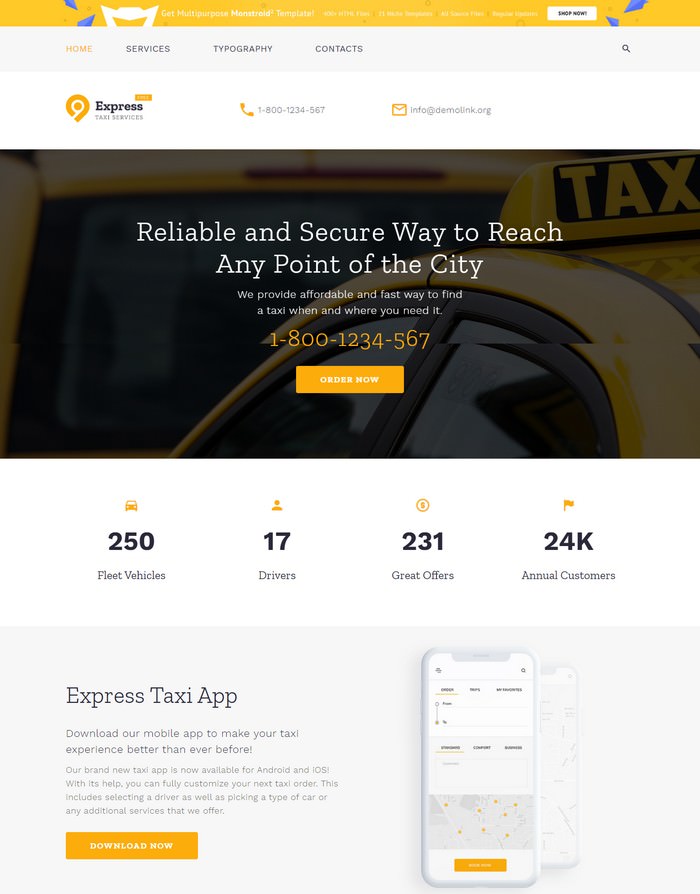This image showcases the homepage of the "Express" website. Dominating the upper portion, a yellow bar spans horizontally from left to right, featuring the "Express" logo—a yellow pinpoint emblem. Below this bar is a gray horizontal menu bar. Menu options such as "Home," "Services," "Topography," and "Contact Us" are clearly listed from left to right.

Directly beneath the menu bar, the "Express" logo is prominently displayed, accompanied by the company's contact details: a phone number and the email address "info@demolink.org." Below these elements is a banner with a compelling tagline, "A reliable and secure way to reach any point of the city," offering both a contact phone number and a prominently displayed "Order Now" button for immediate action.